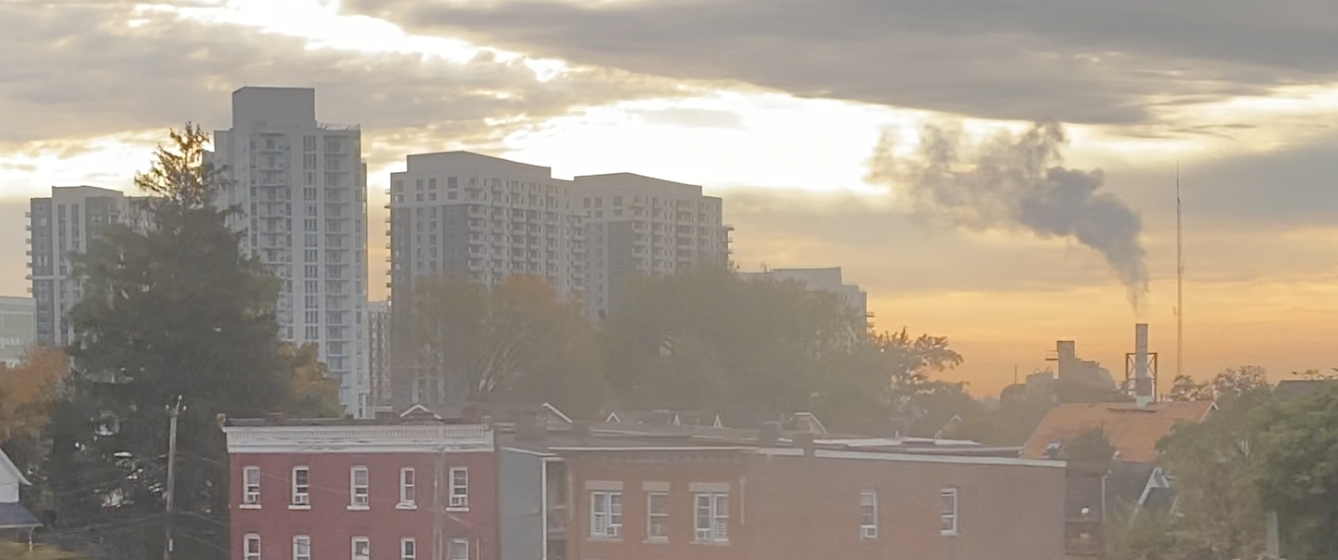This is a photograph of a cityscape under a cloudy, gray sky, either at dawn or dusk, casting shadows across the scene. In the foreground, there are two prominent red brick apartment buildings, roughly three to four stories high, with numerous windows and a couple of trees taller than these buildings. To the right of the apartment buildings, a smokestack from a business emits smoke into the air, contributing to the smog. There is also a tall radio station antenna adjacent to the smokestack. The background features several skyscrapers with multiple floors and balconies, enhancing the urban feel. The scene includes a mix of green and brown trees, but notably, there are no people or animals present in the photo.